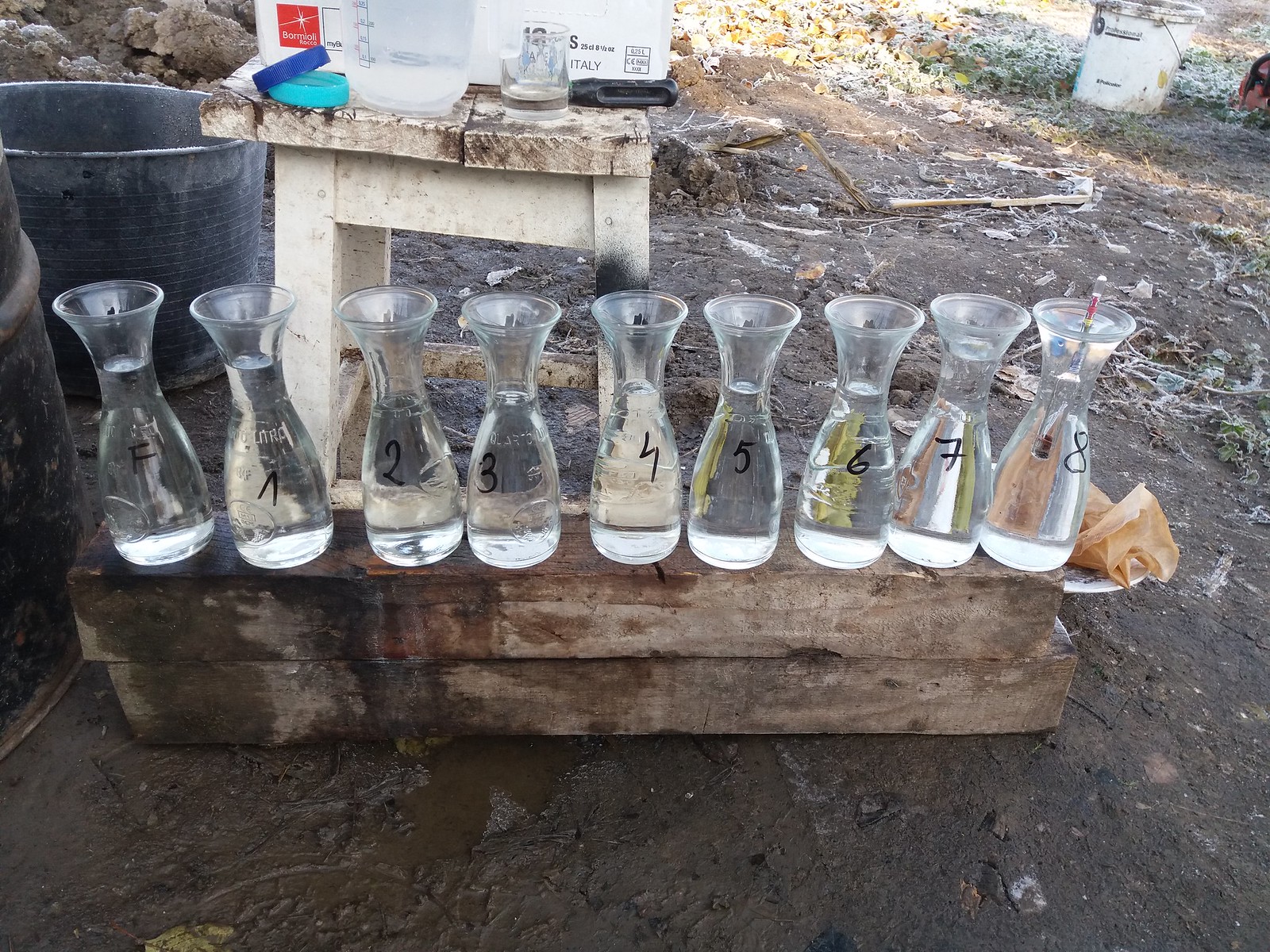This outdoor photograph appears to capture a backyard or a muddy area, possibly part of someone's property or a farmhouse. Featured prominently are nine clear glass vases, each labeled with black marker from 'F' to '8'. These vases are neatly arranged on two horizontal wooden beams. Each vase is filled with water, and the eighth one contains an additional object, possibly a straw, thermometer, or an atmospheric pressure instrument, indicating some form of experimentation. The setup suggests a methodical layout, possibly for a chemical or scientific experiment. In the background, there is a table laden with various equipment, including a large jug, a small glass, a bucket with measurements, and a box marked "Insanity," contributing to the sense of an active work area dedicated to mixing or analyzing substances. The staging in a natural and somewhat unkempt outdoor environment adds a rustic element to the scene.